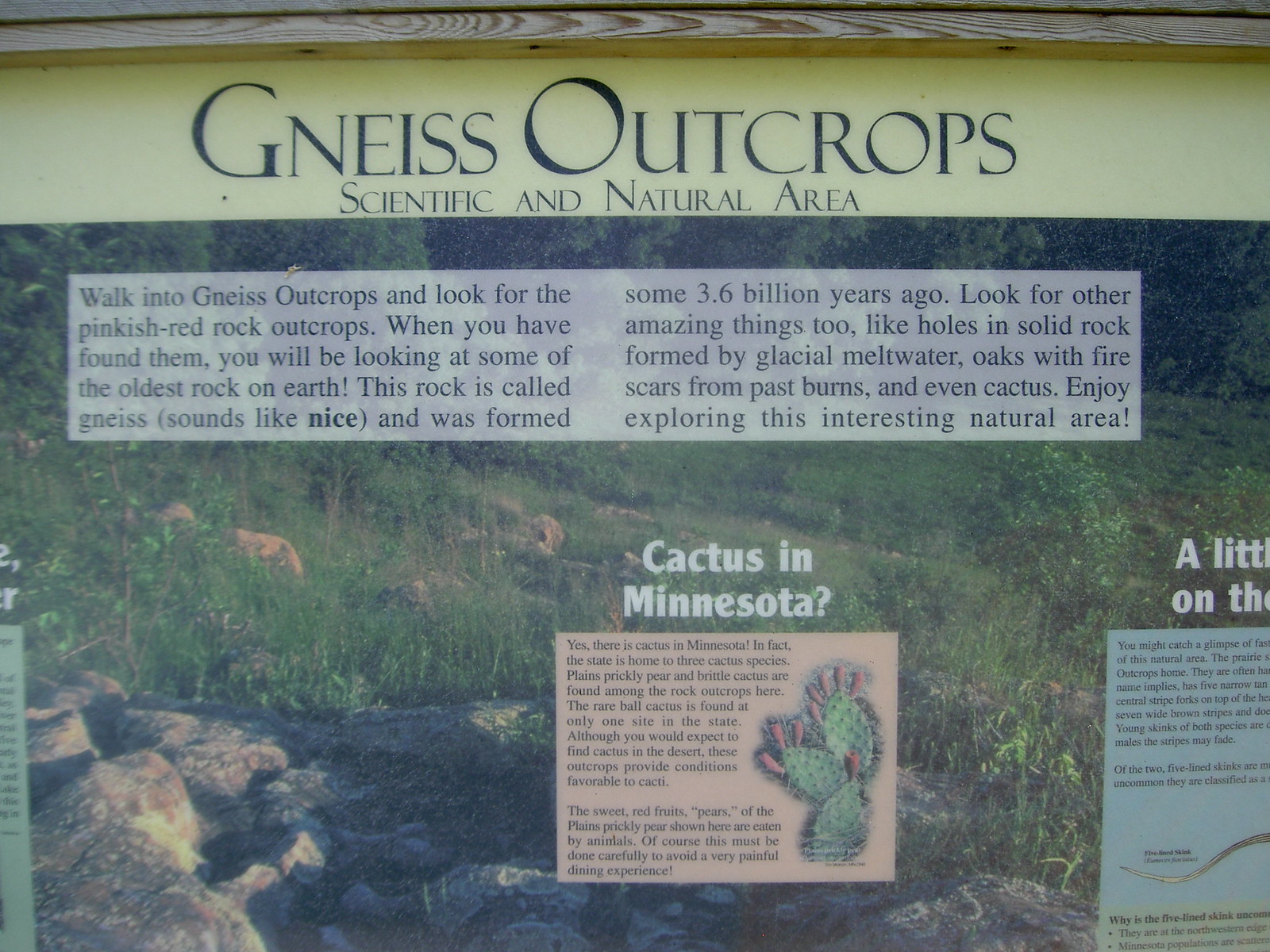The photograph captures a sign for an outdoor scenic area known as "Gneiss Outcrops," distinguished by its yellow top bar with the title in bold black letters. Below it, the sign informs visitors that this is a scientific and natural area filled with lush green vegetation and ancient rocks. Visitors are invited to "walk into Gneiss Outcrops and look for the pinkish-red outcrops." These outcrops represent some of the oldest rocks on Earth, formed approximately 3.6 billion years ago. The rock, pronounced "nice," offers more than just a glimpse into geological history; other intriguing features include holes in solid rock caused by glacial meltwater, oak trees bearing fire scars from past burns, and even cacti. A white text box further explains these details, emphasizing the unique ecosystem and encouraging exploration. An adjoining orange square displays two paragraphs of additional information, next to which a green prickly pear cactus with red blooms is visible. The text below the cactus asks, "Cactus in Minnesota?" in a curious tone. The bottom right corner of the image reveals another white square with black text, bordered by a yellow strip at the bottom, with part of another sign visible on the far bottom left.